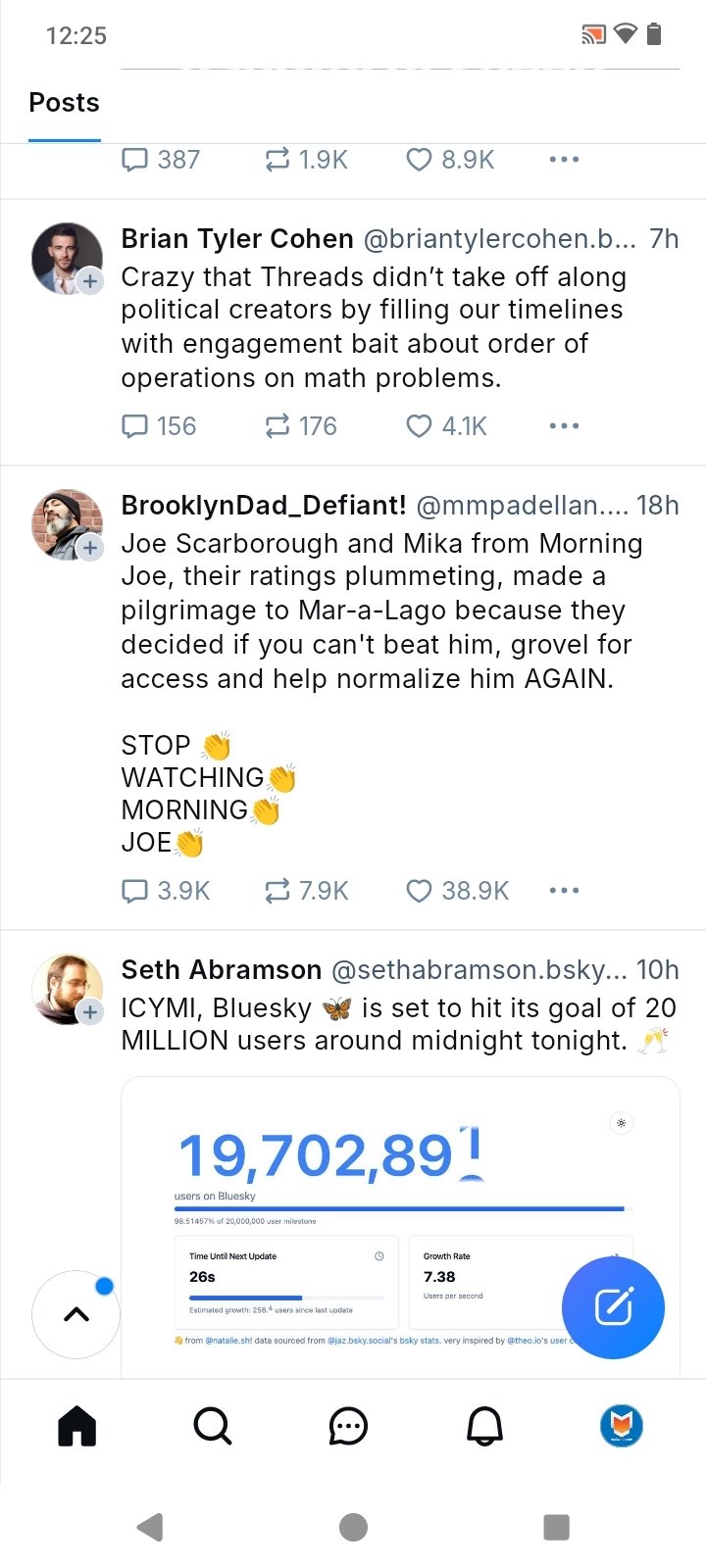Screenshot of a user interface with a black background featuring various settings and account details. On the top left, there's a white left arrow and a settings icon. Below, the account email "malavida.software@gmail.com" is displayed, signed in as "malavida#1 @malavida1.dsky.social." 

Options include:

- **Sign Out:** Displayed in blue text.
- **Add Account:** Accompanied by a gray circle with a plus sign.
- **Invite a Friend:** Displayed with a gray circle and a ticket icon, showing "0 invite codes available."
- **Accessibility:** Featuring a gray circle with an option to "Require alt text on images."
- **Appearance:** This setting has options for "System," "Light," and "Dark" themes, with "System" highlighted in white.
- **Advanced:** Includes "Home Feed Preferences."

There are icons at the bottom representing different sections: a house, a magnifying glass, a semicircle with two lines on top (resembling a rainbow), a mushroom, and finally, a blue circle with an orange badge.